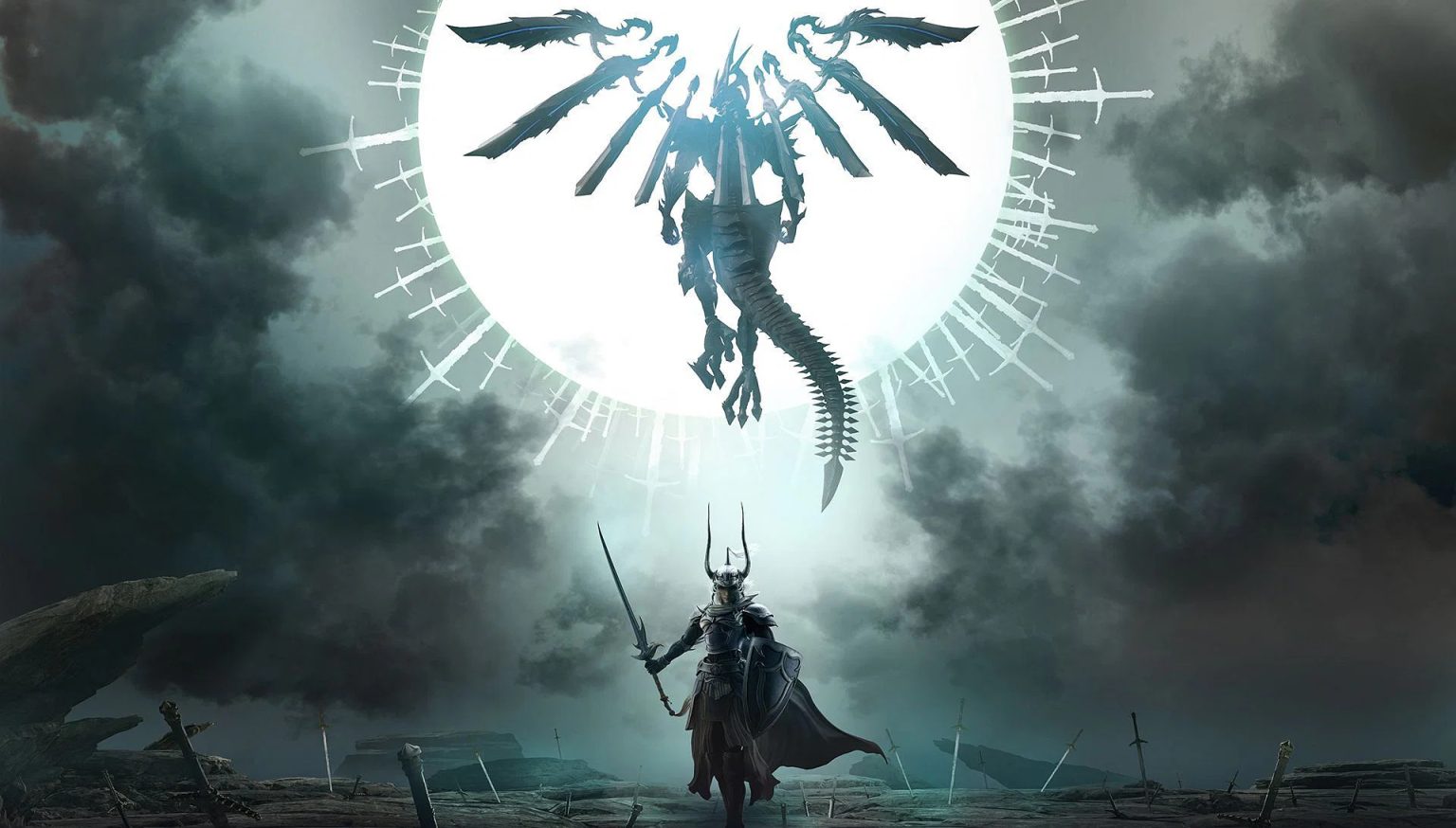The image depicts a dramatic, fantasy scene set in a dark, cloudy environment that appears to be a rocky canyon. Dominating the sky is a dragon-like creature with a skeletal tail, clawed feet, and a bone-like helmet. This creature has numerous swords attached to its shoulders, forming a half-circle around it, and it floats ominously in front of a large, white moon. The moon itself strikingly has multiple swords protruding from it, adding to the surreal atmosphere. Below, a heavily armored warrior stands poised, equipped with a metal helmet adorned with two tall horns, a shield, a long sword, and a flowing cape. The setting and characters suggest an impending epic battle, reminiscent of a scene from a fantasy movie, anime, or video game, lending a heightened sense of anticipation and otherworldly tension to the image.